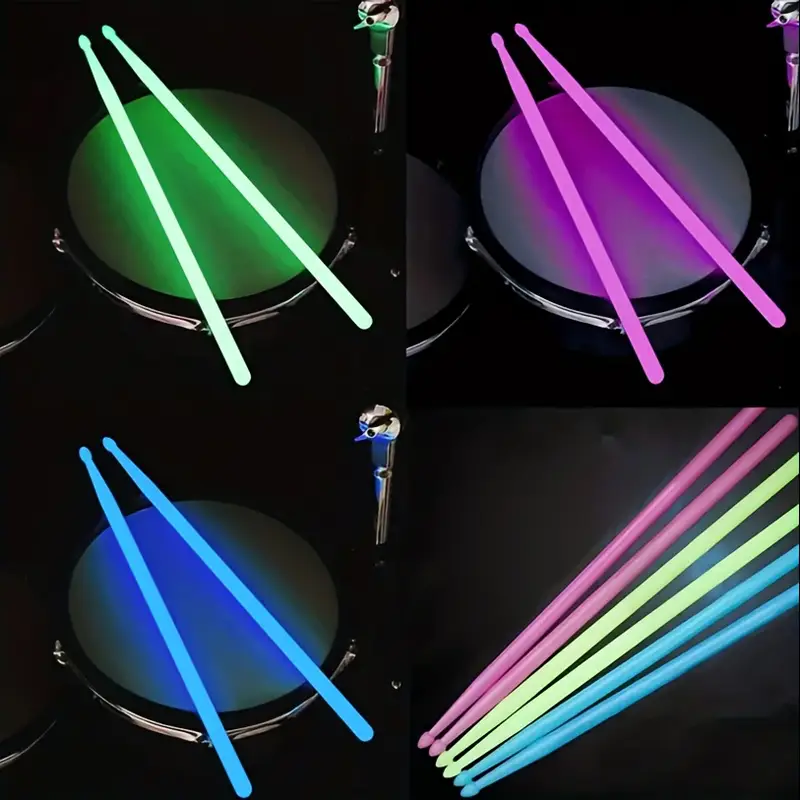This image features a composite of four distinct sections, forming a larger square, each with a dark background to highlight vivid, neon-lit elements. The top left section showcases a drum illuminated with a green light, complemented by matching green drumsticks. In the top right section, a drum glows under a purple light, accompanied by purple drumsticks casting shadows. The bottom left section exhibits a drum lit in blue with a pair of blue drumsticks resting on top. The bottom right section diverges slightly, displaying three sets of drumsticks in vibrant colors—purple, yellow, and blue—all pointing downward and to the left. These striking neon hues and the dark backdrop emphasize the fluorescent glow of the drums and drumsticks.